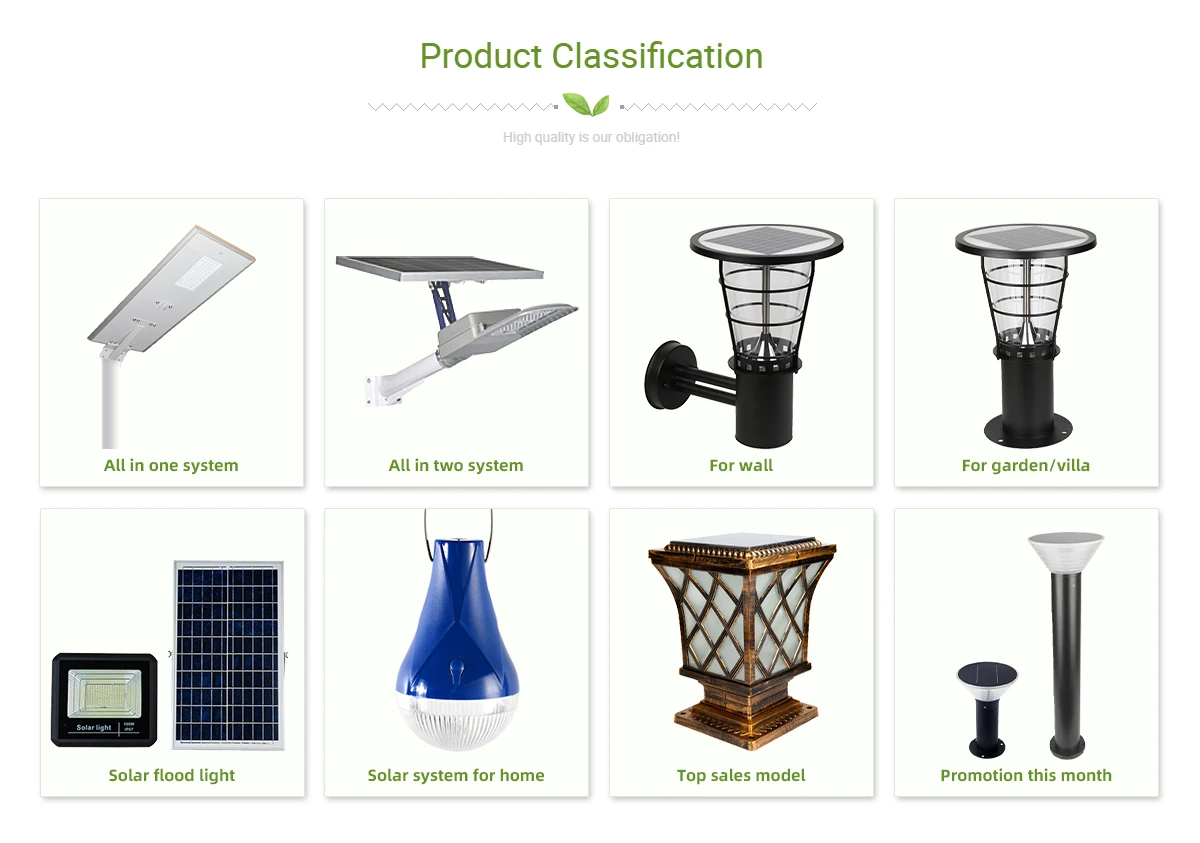This image displays a section of a website with a clean, white background featuring two rows of four images each. At the very top of the page, "Product Classification" is prominently displayed in green text, accompanied by a decorative green squiggly line with two green leaves in the center. Just below this design, a light gray phrase reads, "High quality is our obligation."

In the top left corner, there is an image of a product labeled "All-in-One System," which appears to be a rectangular light mounted on a metal pole. To the right of that, another product called "All-in-Two System" is shown. This one features a flat solar panel on a black bar with a metal arm extending out, ending with a silver light fixture.

Continuing to the right, the next product is a black lantern-style light designed for wall mounting, labeled "For Wall." Adjacent to it, another black lantern is displayed, which is described as being suitable for a "Garden Villa."

In the bottom row, starting from the left, there is an image of a product called "Solar Floodlight," which consists of a small square light paired with a larger rectangular solar panel. To the right, an item labeled "Solar System for Home" is depicted, featuring a distinctive raindrop-shaped light with a blue top and white bottom section.

Next in line, a lantern with a copper finish, showcasing a diamond pattern, is labeled "Top Sales Model." Finally, on the far right, there is a torch light identified as being on promotion for the current month, carrying the descriptor "Promotion This Month."